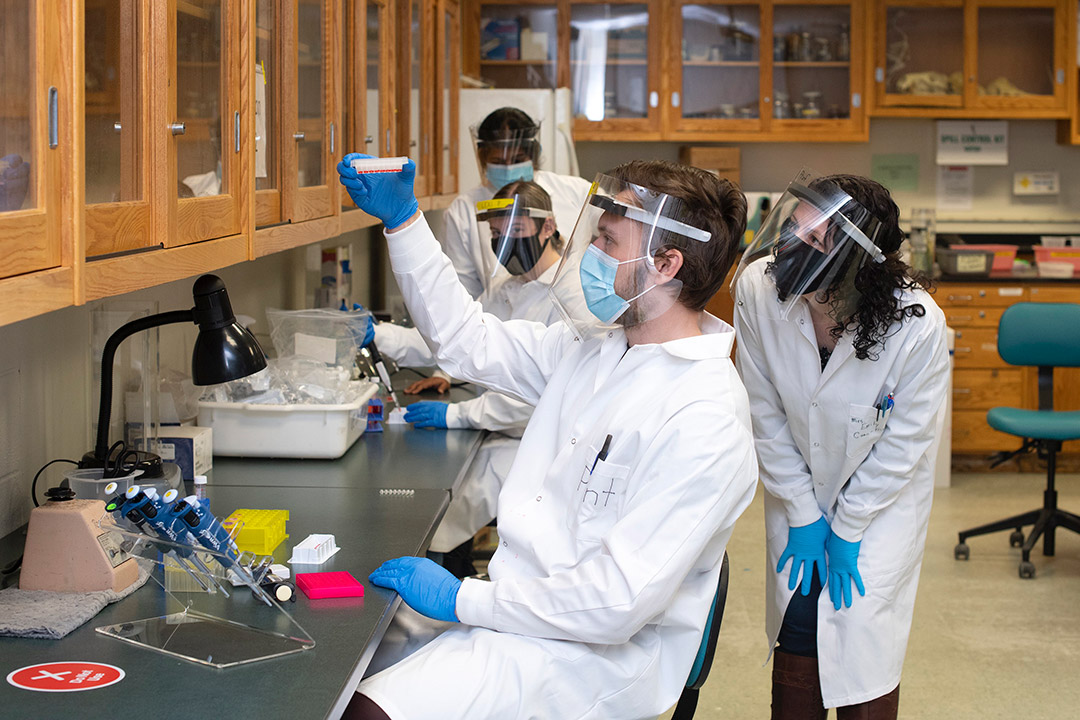In a bustling laboratory, four scientists—two females and one male—are conducting an experiment. Clad in white laboratory coats, blue latex gloves, surgical face masks, and plastic face shields, they are intently focused on their task. The main attention is on a male scientist with short brown hair who is holding up a petri dish and examining its contents. A female scientist with long black hair, crouching closely behind him, peers over his shoulder to observe the petri dish as well. In the background, two more female scientists are conducting their own pipetting experiment but are also glancing toward the petri dish. The laboratory, reminiscent of a biology classroom, features glass-covered cabinets and a blue chair situated in the middle of the room. Several hazard warning signs on the counter emphasize safety precautions.